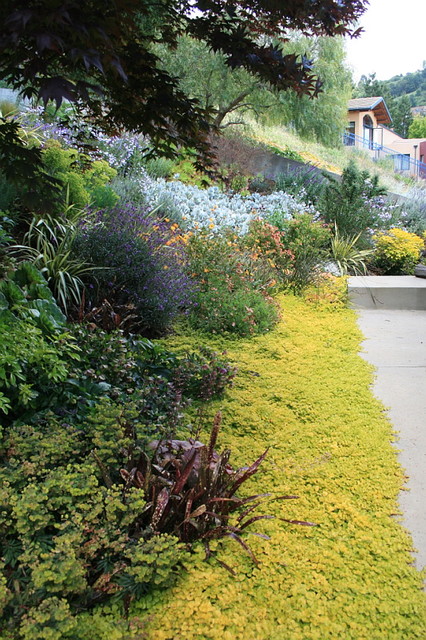The image captures a beautifully landscaped outdoor scene dominated by lush vegetation. The right-hand side of the image reveals a small section of concrete pavement, partially overrun by a yellowish-green ground cover resembling adjuga. Central to the image is a striking plant with purplish, upright, spiky leaves. The background teems with masses of flowers in a vibrant mosaic of purple, white, peach, orange, yellow, and blue hues, all nestled amongst various shades of green foliage. Overhead, the arching branches and leaves of a majestic red Japanese maple create a natural canopy. In the far right background, a light beige house with windows and a handrail sits atop a hill, anchored to the scene by a stone path that intersects this verdant paradise. The composition of verdant ground cover, diverse flowering plants, and the overarching trees crafts a picturesque, highly detailed garden.